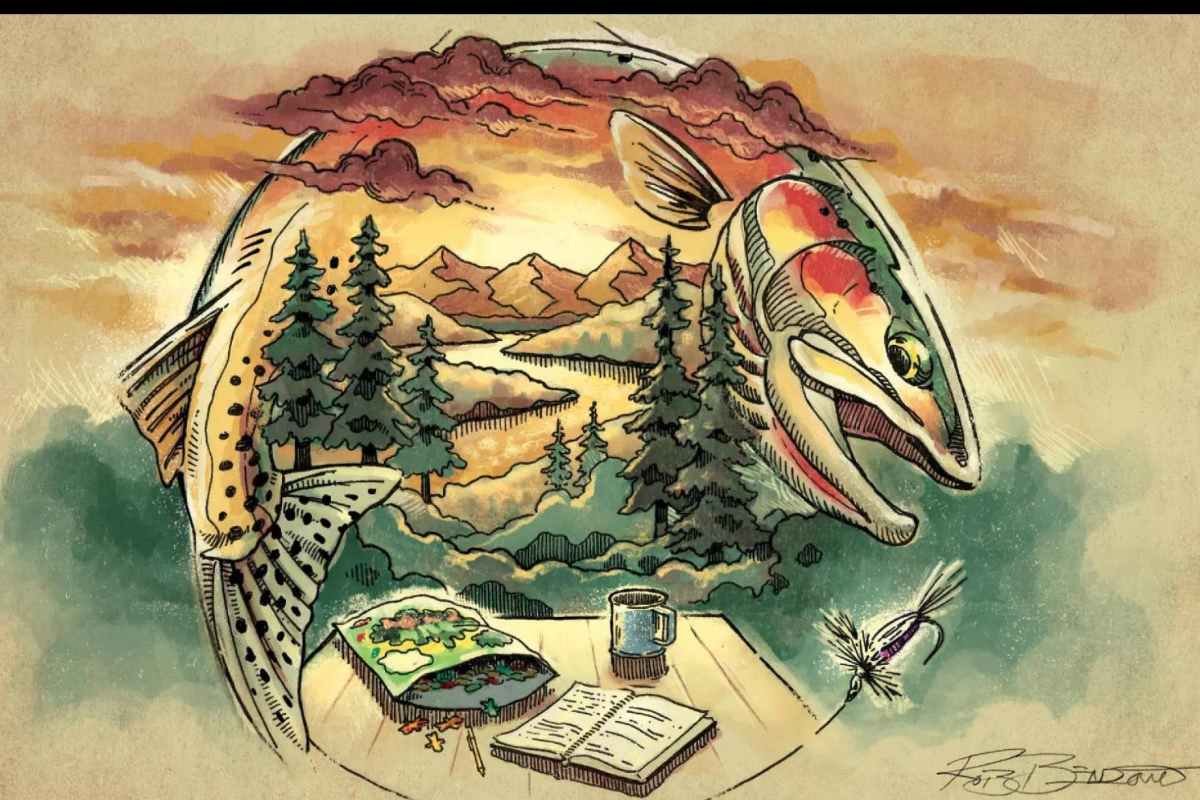The image is an abstract painting prominently featuring a fish with colors ranging from green, yellow, red, and brown, arranged in a semi-circular form that encloses a vivid landscape scene. The fish's head appears on the right, with its tail curling to the left, forming a circular space. Above the fish, the sky is depicted in hues of orange, yellow, and brown, with red clouds forming part of this abstract sky. Inside the circular form created by the fish’s body, there is a detailed landscape with pine trees, hills, and mountains against the backdrop of a river and the sun.

In the foreground, the bottom section of the painting shows a wooden table with various items: an open book, a pencil, a blue mug, and a bag of gummy bears or food items. The artist's signature, beginning with an 'R', is visible in the bottom right corner. The painting predominantly employs a color palette of green, yellow, red, brown, blue, orange, and touches of pink and black, showcasing a blend of natural and imaginative elements.